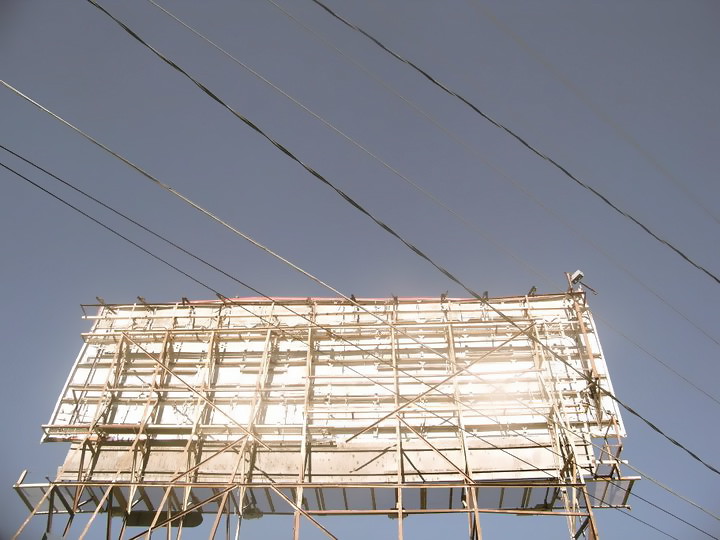An industrial scene under a gray sky, where a network of utility wires crisscrosses the area, creating a chaotic web of lines. In the foreground, the back of a white billboard stands prominently, supporting weathered legs that hint at its age and exposure to the elements. The background is filled with a complex grid of intersecting bars and lines, lending an intricate, almost labyrinthine texture to the composition.